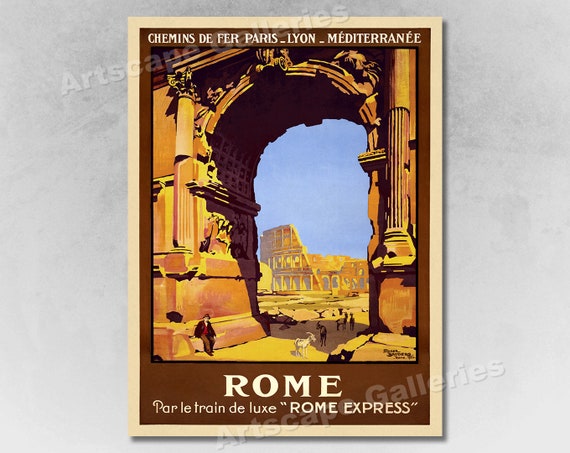This image is a vintage travel poster advertising train travel to Rome. The poster, illustrated rather than photographed, prominently displays the text "Rome par le train deluxe Rome Express," suggesting a luxurious train journey to Rome. The top of the poster includes French text "Chemines de Fer Paris Lyon Méditerranée," indicating a tour route starting in Paris, passing through Lyon, and reaching the Mediterranean.

The central illustration features an archway framing the iconic ruins of the Colosseum in the background. A man is depicted sitting at the base of the archway, while several goat-like figures add to the historical ambiance. The color palette consists of varying shades of brown, ranging from dark to rust-colored tones, with a blue hue in the opening of the archway. The poster is bordered with a white outer edge and a light brown inner border, giving it a classic, vintage look.

Additional visual details include two watermarks from Artscape Galleries, indicating ownership rights. The artist's signature is present in the lower right corner, though it is too small to decipher.